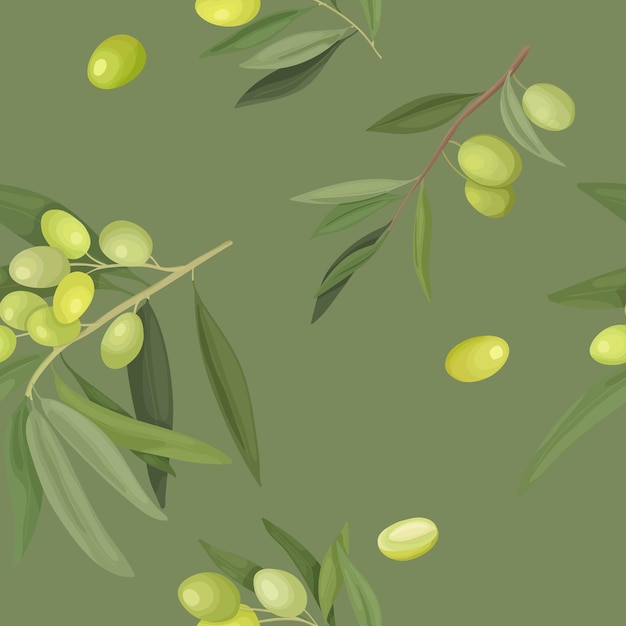The image depicts a segment of wallpaper or a fabric textile with a primarily dark green, almost army green, matte background. The design features detailed branches of what appear to be light chartreuse to mint green olives or possibly green grapes, accompanied by slender, dark green leaves. The branches are woody and give a floating illusion in the space. There are at least three distinct branches fully visible with additional branches partially cropped at the edges. The olives/grapes have a three-dimensional appearance enhanced by shadowing and subtle light reflections, adding small circles of white to indicate where light hits them. The overall artistic style is smooth and flat, possibly hand-painted or digital, contributing to its elegant and refined texture. This intricate design would make for an appealing wallpaper in a home or could serve as a sophisticated pattern for fabrics and textiles.